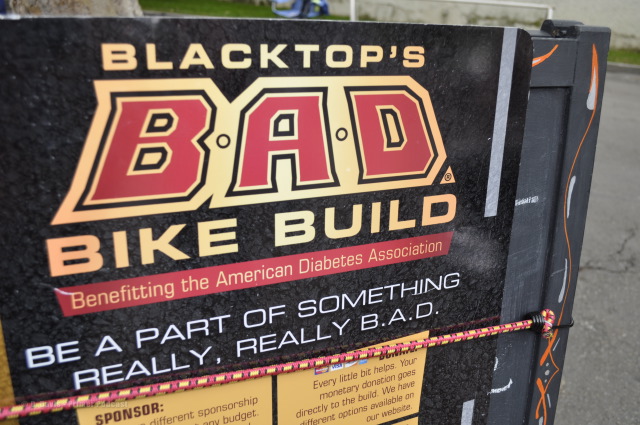The image features a photograph of a banner, seemingly attached to a gate or fence, held in place by a distinctive red and yellow patterned bungee cord. The banner itself has a black background with eye-catching gold and red lettering. The top of the banner reads "Black Tops BAD Bike Build," where the word "BAD" stands out prominently in red letters with a gold outline, further encircled by black, with small circles separating the letters.

Below the main headline, the banner states, "Benefiting the American Diabetes Association," followed by the slogan, "Be a part of something really, really B.A.D." Additional informational sections on the banner mention sponsors and ways to donate, though some of this text is partially obscured by the bungee cord. The banner also emphasizes that "Every little bit helps," indicating different donation options available on a website. The setting appears to be outdoors, with visible street and grassy background elements.